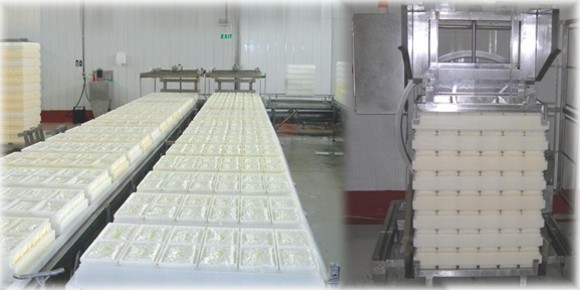The image depicts a sterile and clinical-looking factory interior, characterized by its gray walls and shiny, stainless steel surfaces. Extending from the foreground to the back of the room are multiple long, silver metal tables or conveyor belts laden with neat rows of white plastic trays. Each tray is divided into six smaller square compartments, though the precise contents remain indistinct. On the right-hand side of the image, there is a complex, stainless steel machine with a door-like structure and black handles, possibly part of the production process. Stacked trays of similar white squares extend upward on a metal rack adjacent to the machine, which stands against a wall with a small window near the top. The scene is devoid of human presence, emphasizing the automated, orderly nature of this production line.